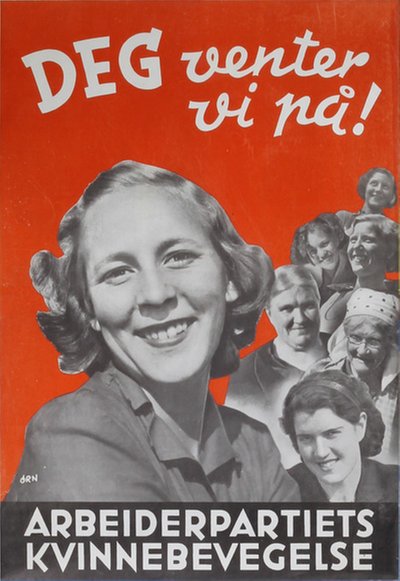The image appears to be an old poster or magazine cover, likely from the 1950s, featuring a prominent black-and-white photograph of smiling women. The background is predominantly red, adding a striking contrast to the monochromatic photos. At the top, in white text, appears the phrase "D-E-G Venter Vi N-C-I!" or a similar sequence, indicating foreign language content. The central figure is a woman with short, curly, dirty blonde hair, wearing a dark-colored collared shirt, standing out among the smaller profiles of other women behind her, who also look directly at the camera and smile. At the bottom of the poster is a black horizontal band with more white text, including a long word starting with "A" and ending with "S," likely "Arbeiderpartiets," and below it, a similar lengthy word starting with "K," possibly "Kvinnebevegelse."